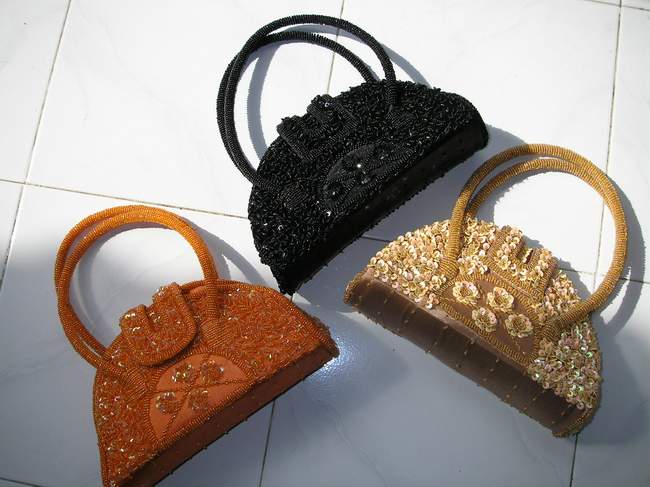The image showcases a trio of small handbags meticulously arranged side by side on a white tile floor, illuminated by a warm daylight glow. Each handbag has a distinct color: the one on the left is a beaded orange, the one in the middle at the top is black and also beaded, and the one on the right is a golden color with a sequin and stitch design. Despite their color differences, the handbags share the same design—they all feature two ruffled handles and a decorative pattern at the base, which consists of four flowers arranged in a cross pattern amidst intricate texturing that gives the bags a floral-like appearance. The careful arrangement and warm lighting highlight both the similarities and subtle differences among the three handbags.